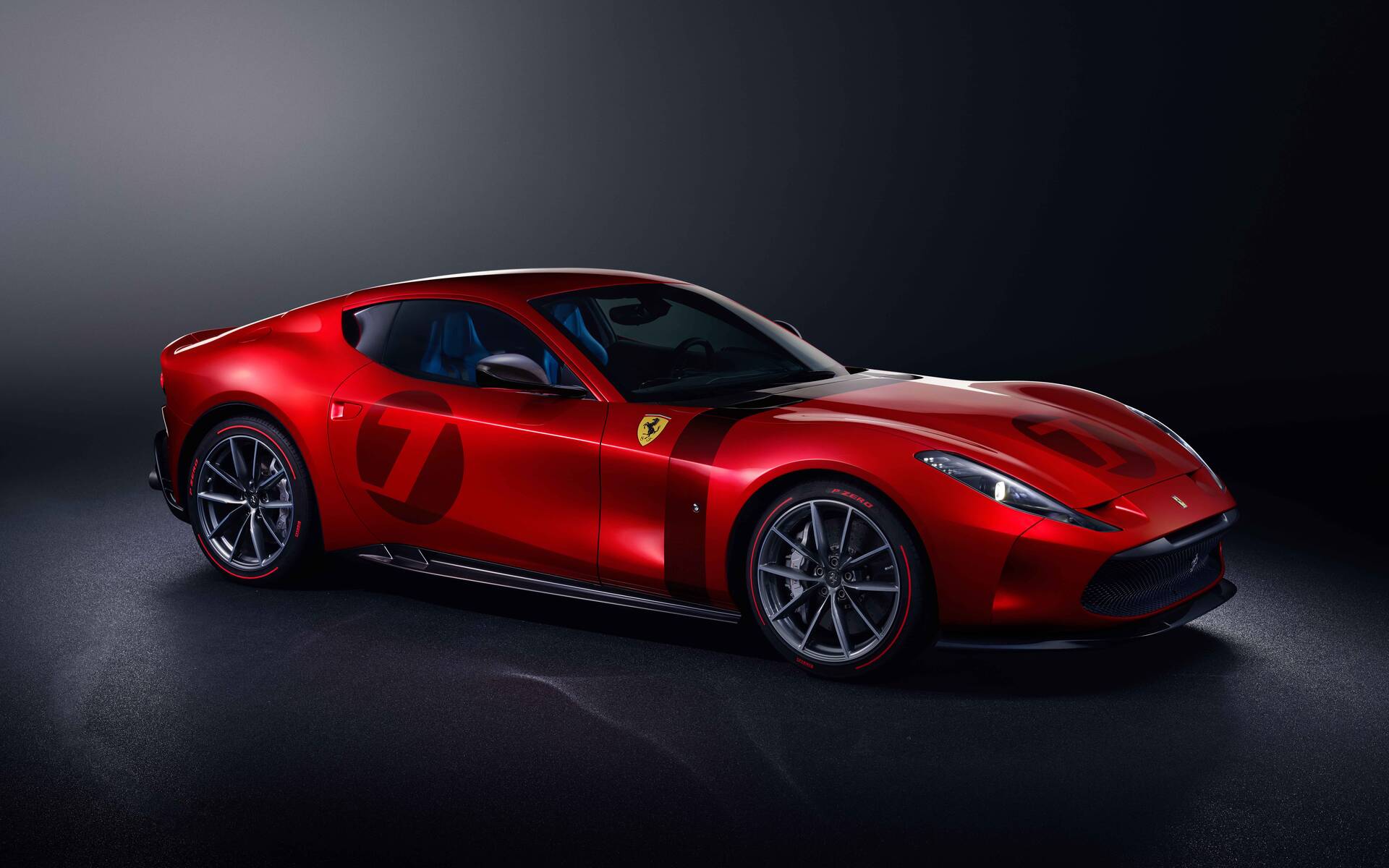The image showcases a striking red Ferrari sports car, captured from a side angle, facing to the right. This sleek, low-slung vehicle features prominent silver wheels with black tires accented by a red rim. The car's number "7" is displayed in a bold circle on both the door and the hood, with illuminated lines extending towards the wheels. The exterior boasts a polished deep red hue, while the interior seats appear to be a shade of blue. The background is a dark gray, almost black, which dramatically highlights the car's vivid color and sleek design. No text is present in the image, allowing the viewer to focus entirely on the Ferrari's elegance and detail. Additionally, there seems to be a yellow and brown detail visible near the front left side of the car.